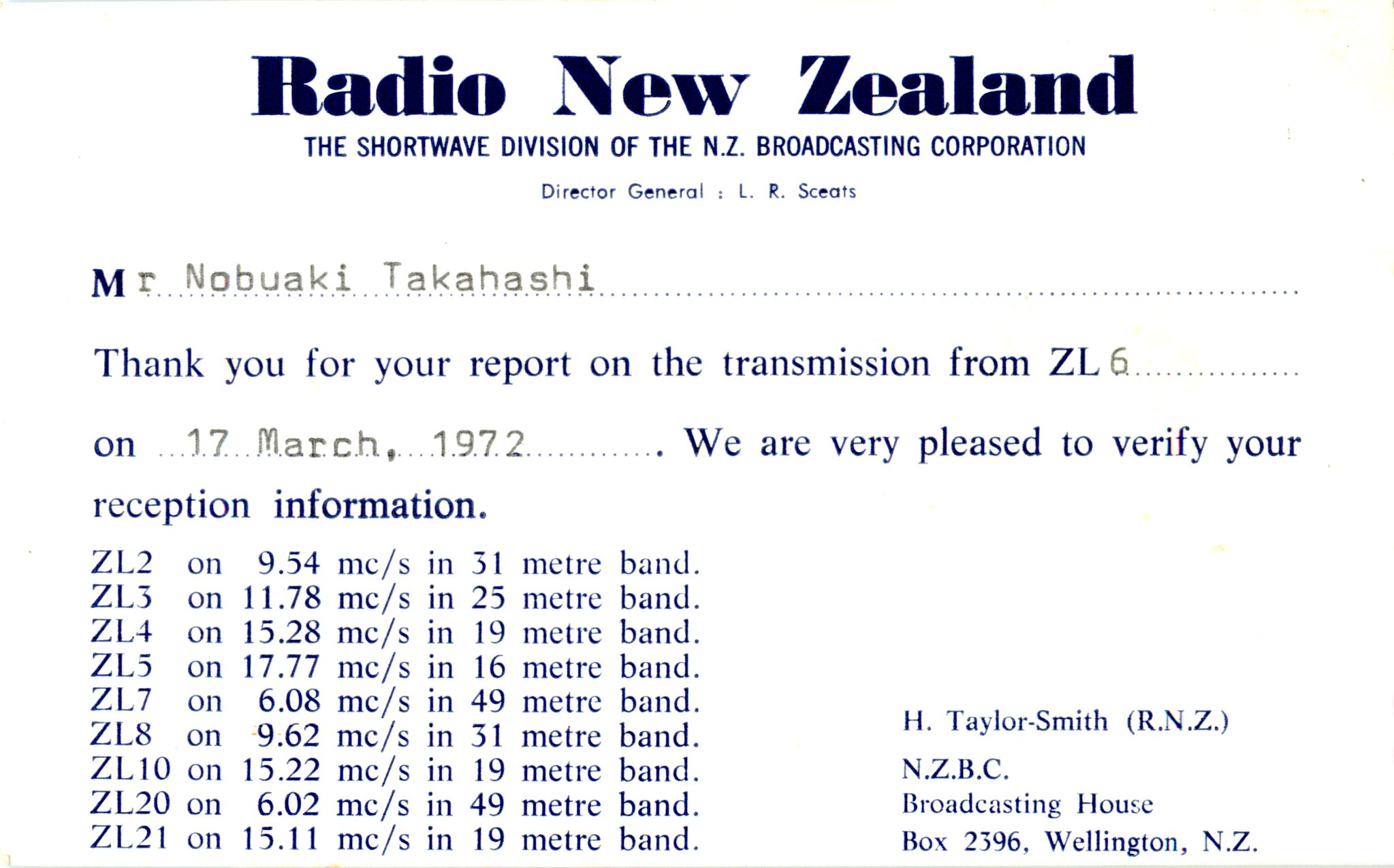The image features a broadcast confirmation receipt from Radio New Zealand. At the top center, "Radio New Zealand" is prominently displayed in large, bold text. Beneath this, in a smaller font, it reads, "The Shortwave Division of the NZ Broadcasting Corporation." Further down, it mentions Director General L.R. Skeets. 

Following this header, the form addresses Mr. Nobuaki Takahashi, thanking him for his report on the transmission from ZL6 on 17 March 1972. The text confirms the receipt and verification of his reception information. Detailed frequency readings are provided: ZL2 on 9.54 MCS in the 31-meter band, ZL3 on 11.78 MCS in the 25-meter band, and ZL4 along with other stations up to ZL21 on various frequencies and meter bands. 

The bottom right corner of the image contains the signature and details of H. Taylor Smith, indicating the formal address: RNZ, NZBC Broadcasting House, Box 2396, Wellington, New Zealand.